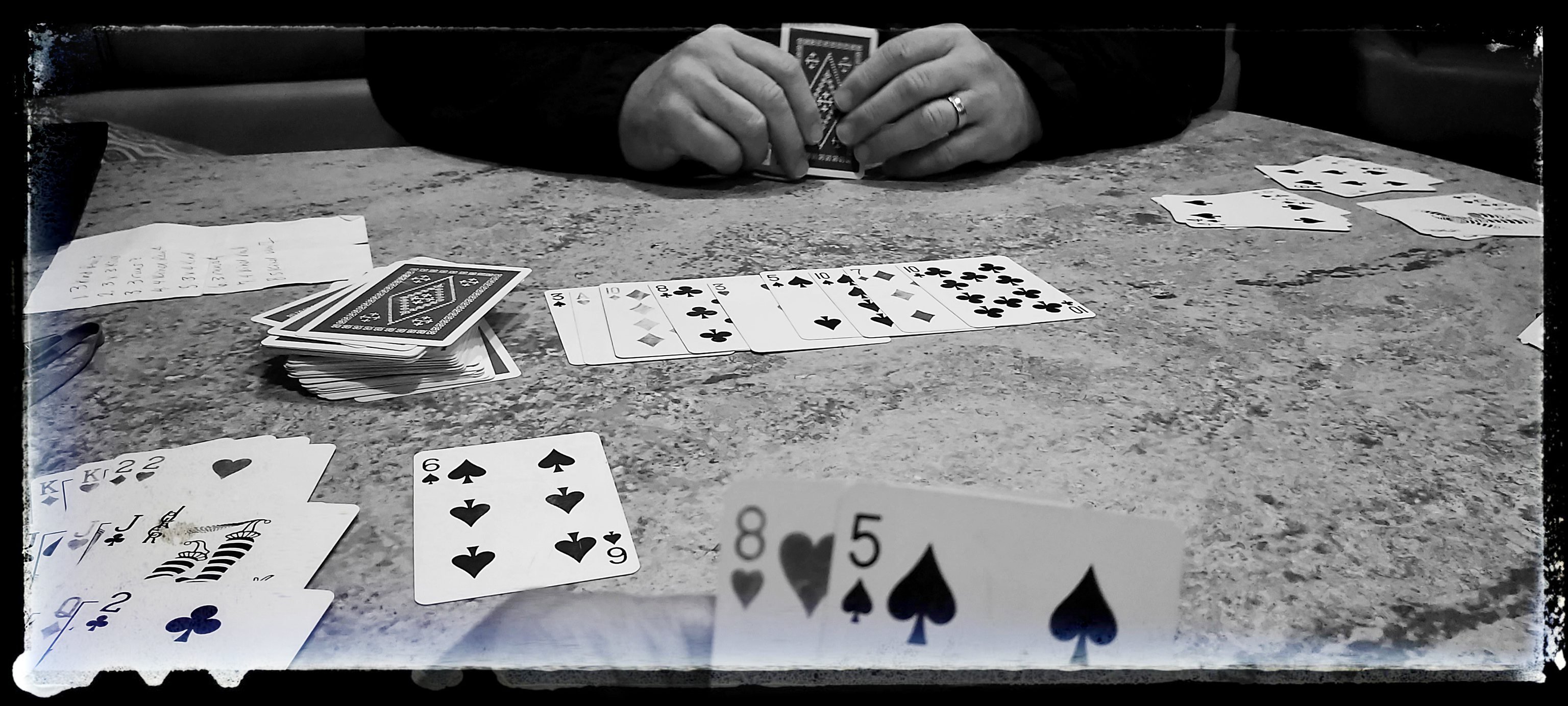In a black and white photograph, a person takes center stage, holding a card adorned with a colorful pattern. Their attire includes black sleeves, and a wedding ring is visible on their hand. To the left, a sheet of paper leans against a notably tall stack of cards, while the right side of the image reveals several scattered cards. Among the cards lying face-up in the middle are a mixture of clovers, spades, and diamonds. Towards the bottom left, a fanned-out array of cards reveals hearts, clovers, and the six of spades. Prominently in the foreground, the person holds the eight of hearts and five of spades. The table beneath them appears to be granite, primarily light-colored with black accents. The image itself is bordered with a frayed edge that fades into a black frame, adding a touch of vintage charm.